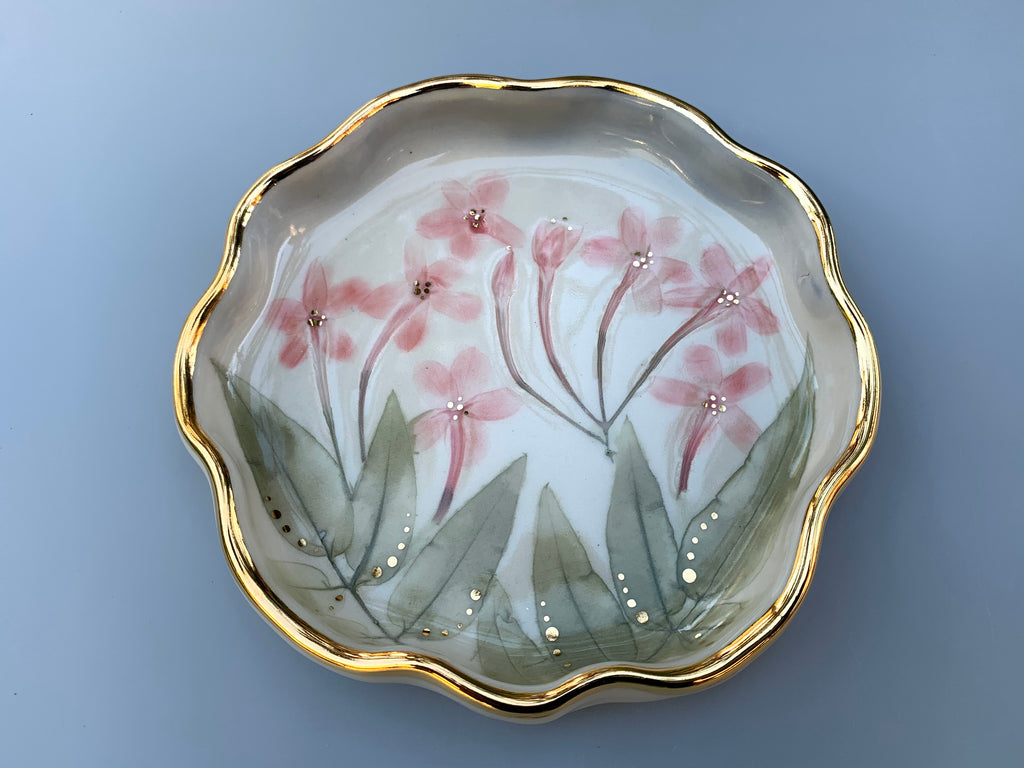In this photograph, a highly polished ceramic dish sits on a light blue tabletop, showcasing its glossy finish that reflects light beautifully. The dish, which appears to be in the shape of a flower with scalloped, curvy edges, features an elegant gold trim that adds a touch of luxury. The main body of the dish is painted in a delicate whitish-gray tone. Adorning the bottom of the dish are green leaves, resembling fern or peach leaves, accented with small gold dots. The top portion of the dish displays a cluster of approximately ten pink flowers, each with five translucent petals and green stems. These flowers also have gold dots enhancing their centers, harmonizing with the gold elements throughout the design.